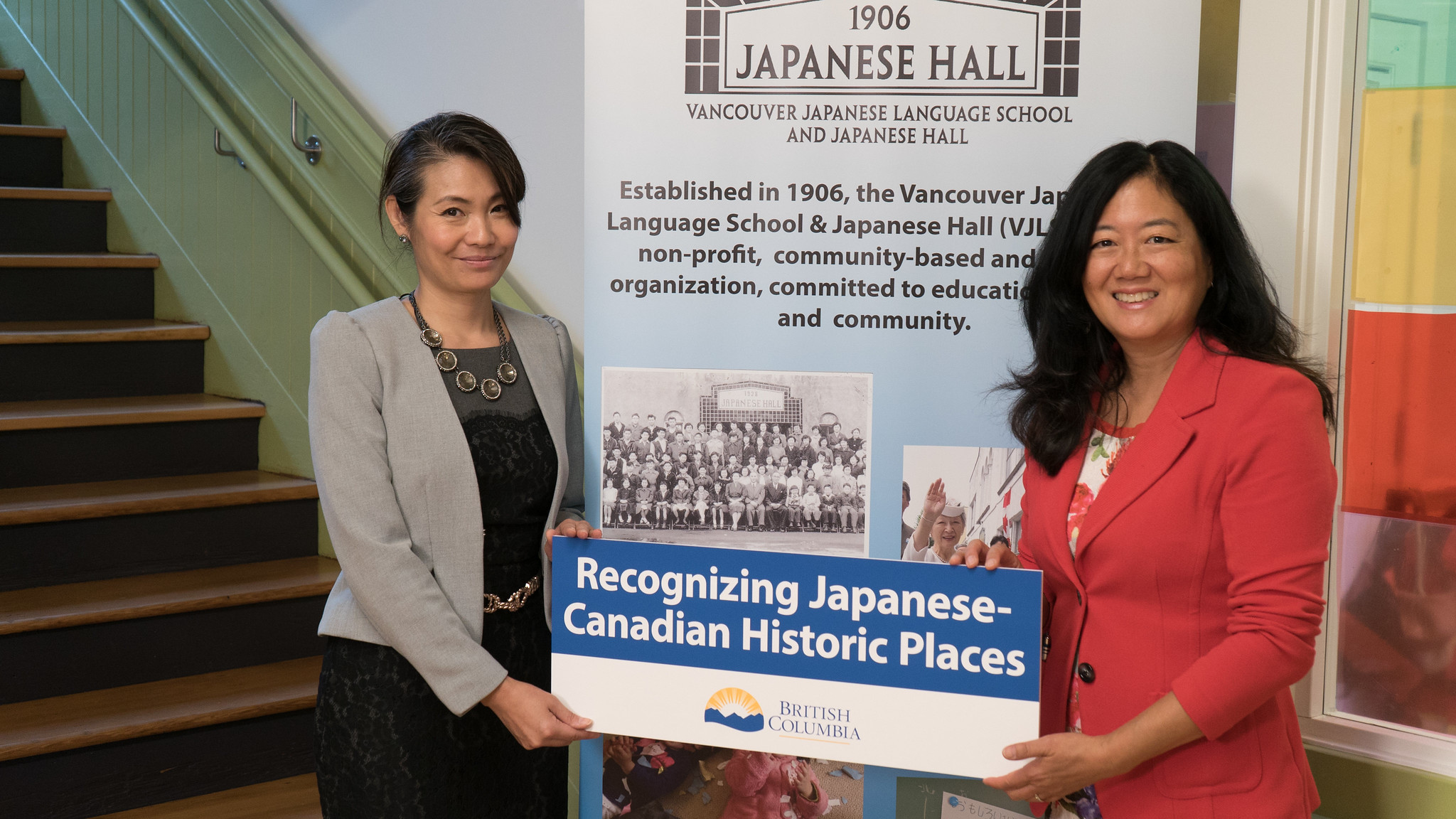In the image, two women stand side by side, holding a sign between them. The top portion of the sign features a blue background with white text that reads "Recognizing Japanese Canadian Historic Places," while the bottom portion is white with a blue British Columbia logo. The woman on the left is positioned in front of a staircase, wearing a black dress complemented by a dark statement necklace, and a light gray blazer. The woman on the right is dressed in a floral print dress and a coral blazer. Behind them, an additional sign with a light blue background bears black text which states: "1906 Japanese Hall, Vancouver Japanese Language School and Japanese Hall. Established in 1906, the Vancouver Japanese Language School and Japanese Hall is a non-profit community-based organization committed to education and community." The setting and attire suggest a formal event recognizing important cultural heritage sites.